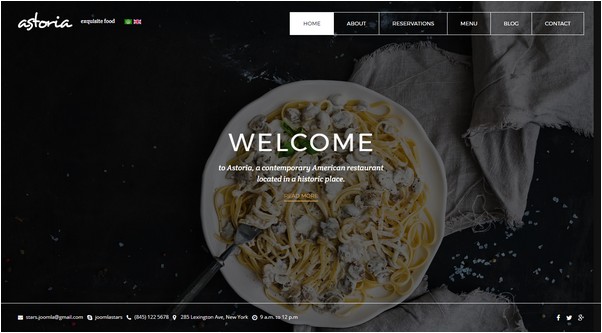The image is a screenshot of a website with a background featuring a high-resolution photograph of linguine pasta in a creamy white sauce, served on a white plate. A fork enters the frame from the bottom left, suggesting a moment just before a bite. The plate rests on a table with part of a cloth, possibly a napkin or tablecloth, visible under the plate and extending towards the top right corner. The image appears to have a dark overlay, reducing its saturation and emphasizing the website's content over the background.

In the top left corner, the word "Astoria" is written in a handwritten-style font, followed by unreadable white text beneath it. The website's navigation bar is positioned along the top right, with several menu options: Home, About, Reservations, Menu, Blog, and Contact. The selected option, Home, has a white background with dark text, while the others feature a dark background with light text and outlines.

The central text of the page prominently displays "WELCOME" in large, all-caps white text. Below it, in italicized letters, is a subheading that reads, "To Astoria, a contemporary American restaurant located in a historic place." A yellow link beneath this text appears to say "Load More." 

At the bottom of the page, a light line is visible with links or contact information that are not fully readable. Additionally, social media icons are aligned along the left and right margins of the page.